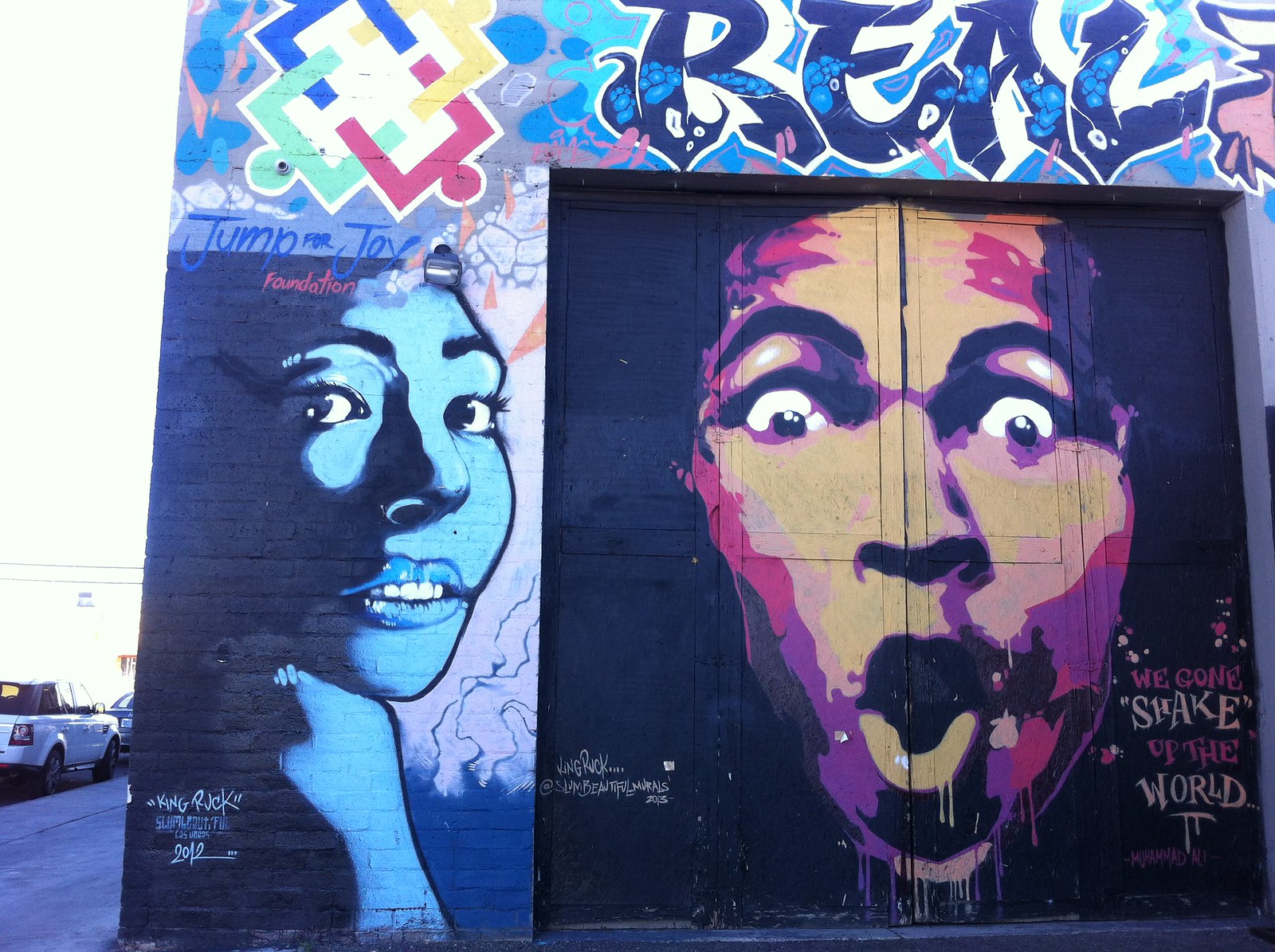The image depicts an outdoor scene captured during the daytime, featuring a detailed street art display on a brick wall and a dark black garage door. The setting includes a stone walkway or sidewalk in the foreground with some parked cars visible on the left side of the image. The focal point of the photograph is the vibrant graffiti art that occupies both the garage door and the adjacent wall.

Starting on the right side, the garage door showcases a striking image of a man's face with wide-open eyes and an open mouth, suggesting a surprised expression. This artwork employs a color palette of tan, black, red, and purple. At the bottom right of this mural, there is text that reads, "We Gone Shake Up the World," with "Shake" highlighted in lighter tan and enclosed in quotation marks. The artist's signature, "King Ruck," appears in the lower left corner of the door.

Above the garage door, "Real" is written in black with blue bubble accents. Moving to the left, the wall features another piece of street art depicting a woman's face rendered in shades of blue and white. This mural is accompanied by text reading "Jump for Joy Foundation" in blue beneath it. Both pieces of artwork prominently display the artist's signature, "King Ruck." The entire scene, surrounded by the muted colors of the stone walkway and parked cars, is set against a gray sky, emphasizing the vivid street art central to the composition.